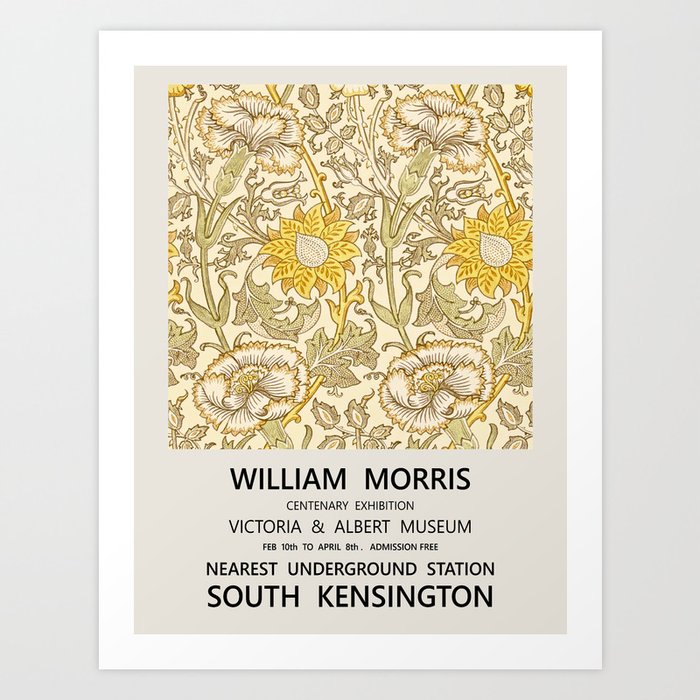This image features a poster against a grayish-lilac background with a white border. Inside the white border, the poster itself has a soft grayish-pink background. At the top part of the poster, there's a simple yet elegant floral pattern on a pink background, featuring illustrations of sunflowers and other flowers in shades of brown, yellow, white, and grayish-green. Below the floral design, the text is presented in black type and reads: "William Morris, Centenary Exhibition, Victoria and Albert Museum, February 10th to April 8th, Admission Free, Nearest Underground Station: South Kensington." The poster promotes an event that took place at the Victoria and Albert Museum in South Kensington, with free admission, and the text is bordered in white at the bottom.